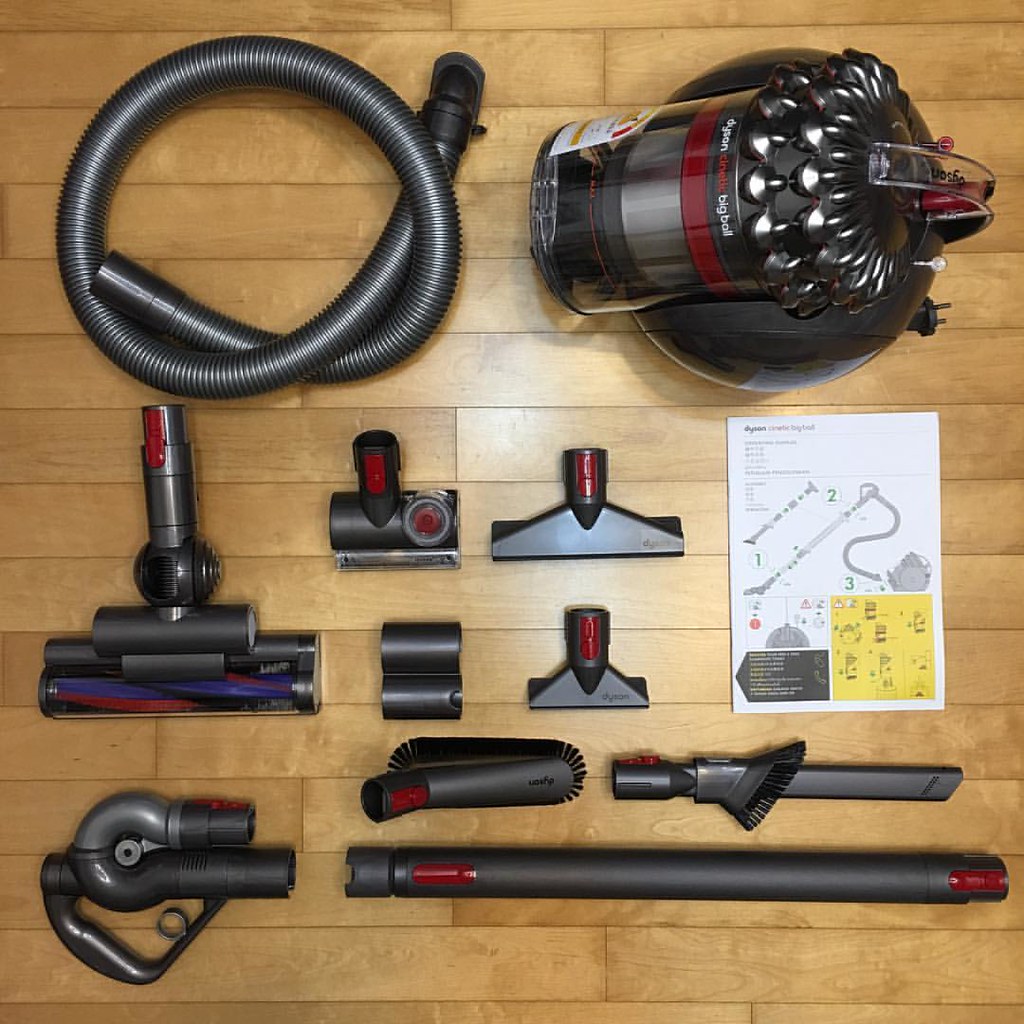This color photograph, taken from an above view, displays a brand new Dyson Big Ball vacuum cleaner meticulously laid out on a light brown, wooden-tiled floor. In the upper left-hand corner, the vacuum hose is coiled like a pretzel, next to the metallic, glossy blackish-gray body of the vacuum with dark red trim. The body prominently features "Dyson Big Ball" in white letters on the top, with an illegible red word between "Dyson" and "Big." The electrical cord's plug is visible to the right of the housing. Neatly arranged below the hose and vacuum body are seven various wands and attachments, aligning in straight and curvy shapes, including small brushes and pieces with a rectangle base. On the right-hand side of the image lies the product guidebook, characterized by white color with dark lettering and numerous illustrations. The overall presentation suggests that the vacuum has just been unboxed, and all its components are organized for assembly.